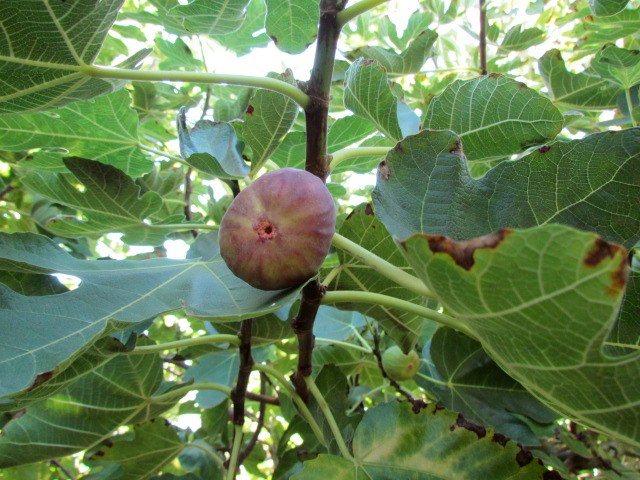In this vibrant and detailed color photograph, a fruit tree stands bathed in bright sunlight with leaves casting intricate shadows. The focal point is a singular, fully-grown fruit situated in the middle of the image, displaying a striking combination of reddish-yellow hues with a pinkish-red circle at its base. The fruit, resembling a donut peach in shape, appears more oblong than round and features unique yellow stripes radiating outward from the center. The leaves, primarily oval with some showing signs of insect activity or sunburn, vary in shades of green, and some exhibit small brown spots. A branch extends from the bottom to the top of the picture, anchoring the fruit and its surroundings. To the bottom left of the main fruit, a smaller, green, and underdeveloped fruit can be seen, indicating it is in the initial stages of growth. The scene lacks a definitive setting but captures the natural essence of a sunlit day with a clear focus on the tree's intricate details.